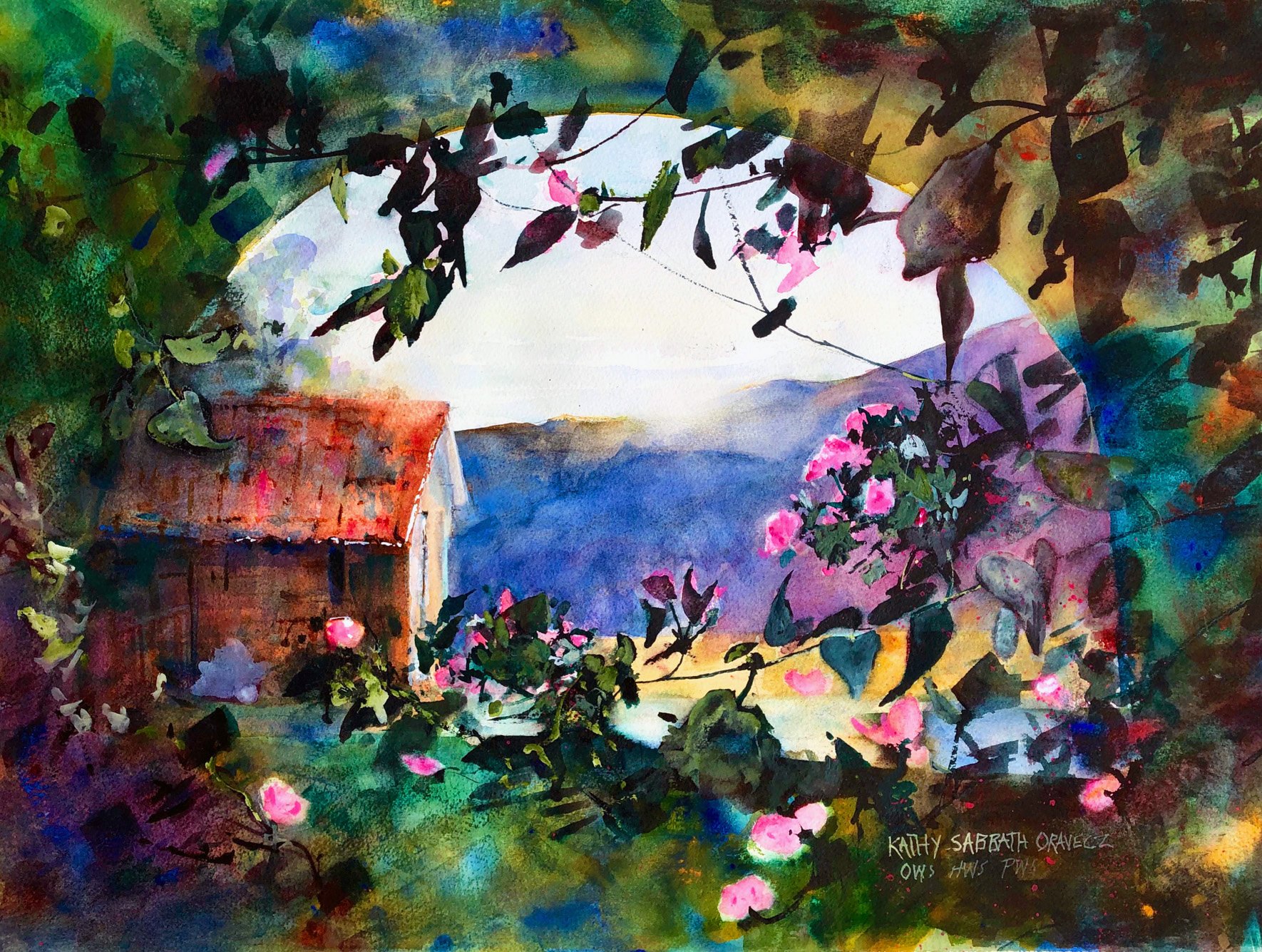This slightly abstract, colorful watercolor painting by Kathy Sabathoravec features a beautiful array of vibrant wildflowers and vines framing a central scene, evocative of looking through a kaleidoscope or a tunnel. The painting’s focal point is a small building resembling a barn with a reddish roof and siding, situated towards the left. The sunlight casts a pale pink hue over the structure. An arch of vines and flowers stretches across the top, creating a natural frame that runs down both sides of the painting. The right side is adorned with lush green leaves and pink flowers, some tinged with white. In the backdrop, watercolor-rendered mountains create a serene horizon, transitioning from bluish and green tones at the peaks to a golden hue at their base. The entire composition is harmoniously intertwined with soft, blended watercolors, lending a slightly abstract and impressionistic feel to the artwork. The bottom right corner of the painting bears the artist's signature.